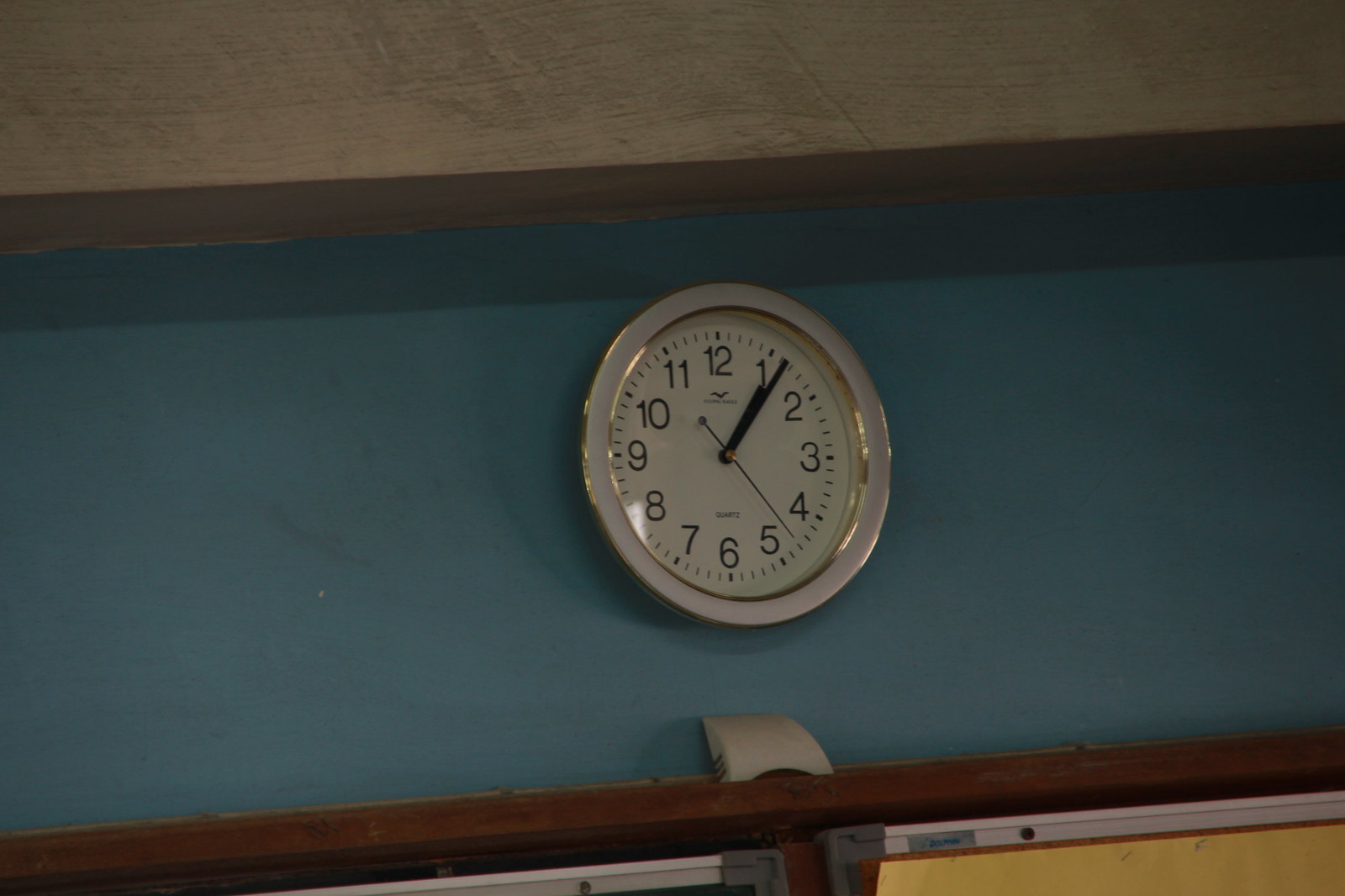A photograph captures an analog wall clock prominently displayed against a blue-gray background, suggestive of an educational setting. The clock, featuring a chrome bezel and equipped with a second hand, minute hand, and hour hand, is situated closer to the ceiling tiles than to the bulletin board below. The ceiling tiles above are striated with patterns of gray and dark gray, adding an aged, textured look to the scene. Below the clock, a seam separates the bulletin board from the upper blue section of the wall, enhancing the sense of an old-school, instructional design. The overall lighting is quite dim, contributing to a vintage, almost nostalgic atmosphere.